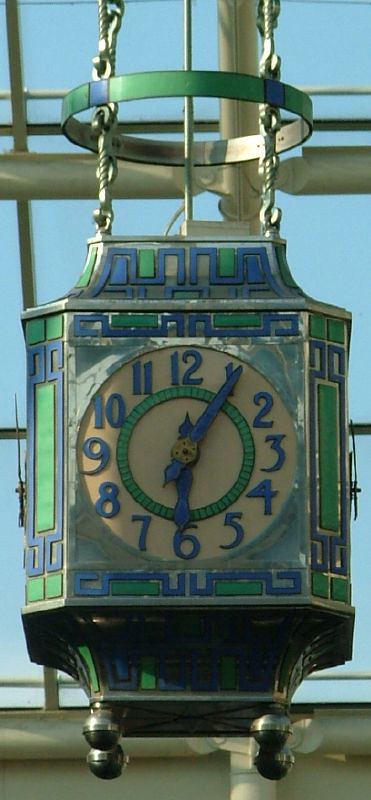This image features a hanging clock set against an outdoor backdrop. The rectangular photograph, with its shorter sides at the top and bottom, captures the clock suspended in mid-air. The background showcases a blue sky accompanied by metal poles used for structural bracing. Chains on either side of the clock and a central gold-hued pole add to the suspension mechanism. Encircling the clock is a circular metal band that is green on the outside and gold on the inside, enhancing its ornate appearance.

The clock itself is predominantly green with blue moldings and intricate rectangular accents on the sides, which feature green centers and blue-green top and bottom details. Trimming the clock is a decorative blue and green border. The clock face, which is round, features a beige background that elegantly offsets the bold, large blue numbers. A green circular trim surrounds the numbers, adding depth to the design. The clock hands are also blue, with their centers highlighted in yellow. At the very bottom of the clock, small gold balls add a finishing touch of elegance.